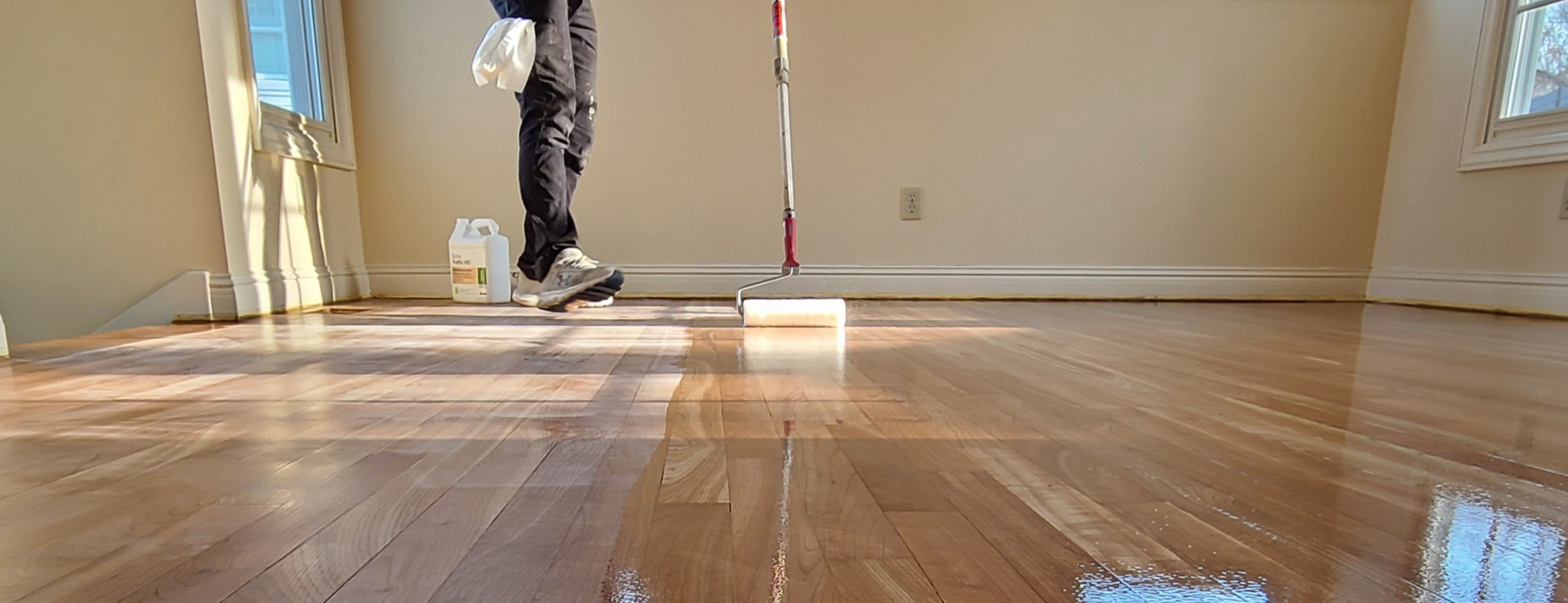The photograph depicts a person waxing or polishing a light-colored hardwood floor. The person is partially visible from the waist down, standing on the left side of the image, clad in dark pants, tennis shoes, with a white cloth tucked into their pocket. In their hand, they hold a long-handled tool with a paint roller on the end, being used to apply the wax or polish solution. On the floor by their feet is a large plastic jug of the solution. The room's walls are painted a light beige or off-white color. The right two-thirds of the floor is already polished, with a stunning shine and visible reflections of light from the windows. The left third remains unpolished, appearing dull and slightly powdery. The image is panoramic and horizontal, capturing the contrast between the polished and unpolished sections of the floor.